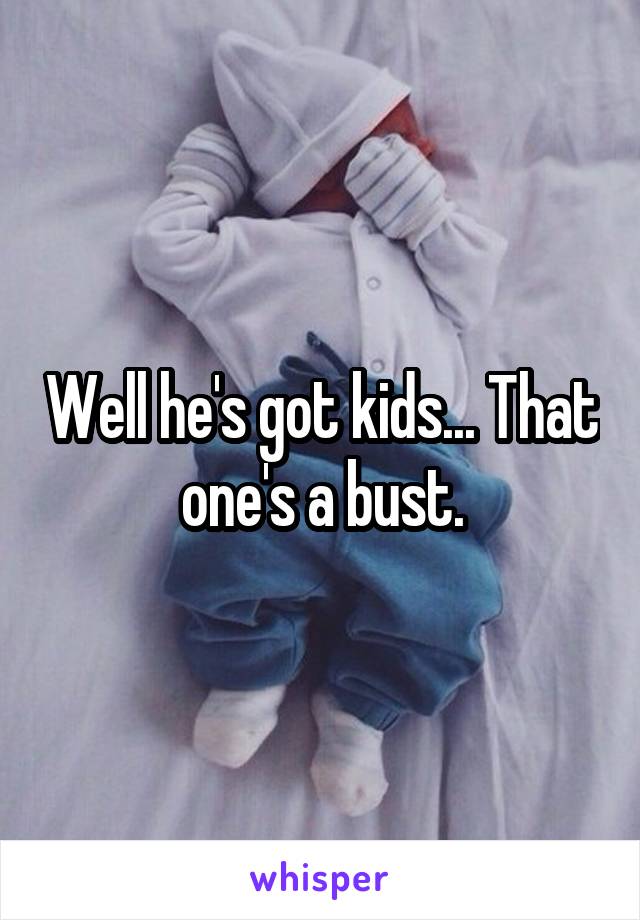The image is a meme featuring a baby dressed in a white hat, white mittens, a white long-sleeve onesie, and blue pants. The baby is lying on a white blanket, with its head turned to the left. The baby's left hand is covering its face while the right hand is positioned behind its head. The picture includes text in white letters with a black outline in the center that reads, "Well, he's got kids, that one's a bust." Additionally, at the bottom of the image, there is a "Whisper" logo in light purple letters, signifying the platform where the meme might have originated. The baby is seemingly asleep, and the photo appears to be taken indoors on a white comforter, adding a cozy and intimate ambiance to the image.